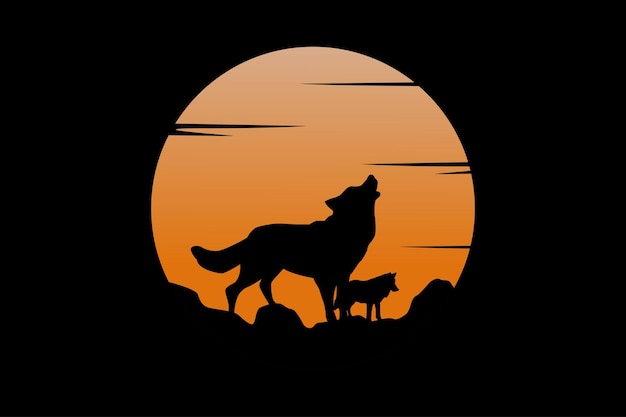The image features a computer-generated artwork set within a wide horizontal rectangle with a stark black background. Dominating the center of the composition is a glowing, light orange circle resembling a moon, which transitions from tan hues at the top to deeper orange shades at the bottom. Encircling the lower edge of the moon are rugged, black, rock-like structures, creating a silhouette. Nestled among these are two wolves depicted in silhouette, their details obscured by the shadows. The larger wolf to the left faces right, its head tilted upward in a howling pose, while the smaller wolf stands more distantly, gazing downward. Several black lines of varying thickness intersect the moon from different angles, adding a layered complexity to the scene. The intricate design with its dynamic interplay of light and shadows evokes a hauntingly beautiful wilderness scene, perfect for transforming into an eye-catching t-shirt graphic.